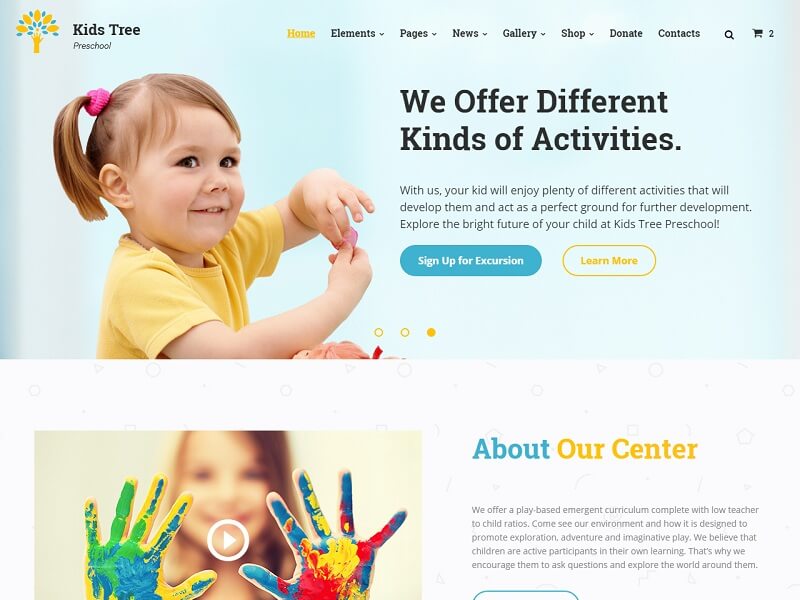The website showcases the homepage for Kids Tree Preschool, prominently featuring an inviting and colorful design. At the top of the page is a navigation bar with links including Home, Elements, Pages, News, Gallery, Shop, Donate, Contacts, and a search icon along with a shopping basket, indicating the capability to purchase items directly from the site. The school's charming logo, a stylized digital icon of a yellow and blue tree, graces the top of the page.

Central to the homepage is a headline that reads, "We offer different kinds of activities," followed by an encouraging message: "With us, your kid will enjoy plenty of different activities that will develop them and act as a perfect ground for further development. Explore the bright future of your child at Kids Tree Preschool." Below this text are two prominent buttons labeled "Sign Up for Excursion" and "Learn More."

Additionally, a section of the about page is visible, describing the preschool's philosophy and environment. It states, "We offer a play-based emergent curriculum complete with low teacher-to-child ratios. Come to see our environment and how it is designed to promote exploration, adventure, and imaginative play. We believe that children are active participants in their own learning. That's why we encourage them to ask questions and explore the world around them."